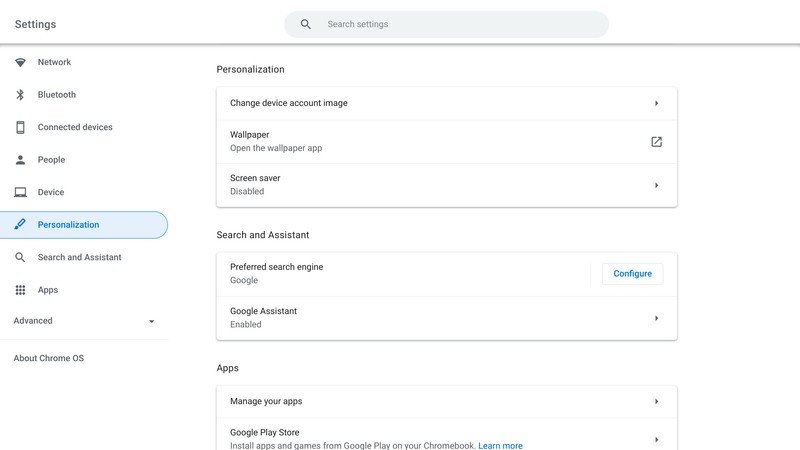This image depicts the settings page of the Google Chrome browser, specifically tailored for Chrome OS on a Chromebook. The page features a minimalist design with a white background, characterized by round-cornered tables and a subdued light gray border. Sections are neatly divided by light gray lines, and there is a subtle drop shadow effect. The predominant text color is a mix of dark gray and black, with blue serving as the accent color.

At the top, a header labeled "Settings" is accompanied by a search bar reading "Search Settings." The interface is divided into two columns: a vertical menu on the left and detailed options on the right. The left menu includes the following sections: Network, Bluetooth, Connected Devices, People, Devices, Personalization (currently selected), Search and Assistant, Apps, Advanced, and Chrome OS. Each menu option is complemented by corresponding icons.

The right-hand column provides detailed settings for each selected section. Under "Personalization," options include "Change Device Account Image," "Wallpaper," "Open the Wallpaper App," and "Screen Saver" (currently disabled). The "Search and Assistant" section features settings for the preferred search engine, which is Google, along with a button to configure it. The Google Assistant is enabled as well. In the "Apps" section, options to manage installed applications are provided, including access to the Google Play Store with a link to learn more about installing apps and games on the Chromebook.